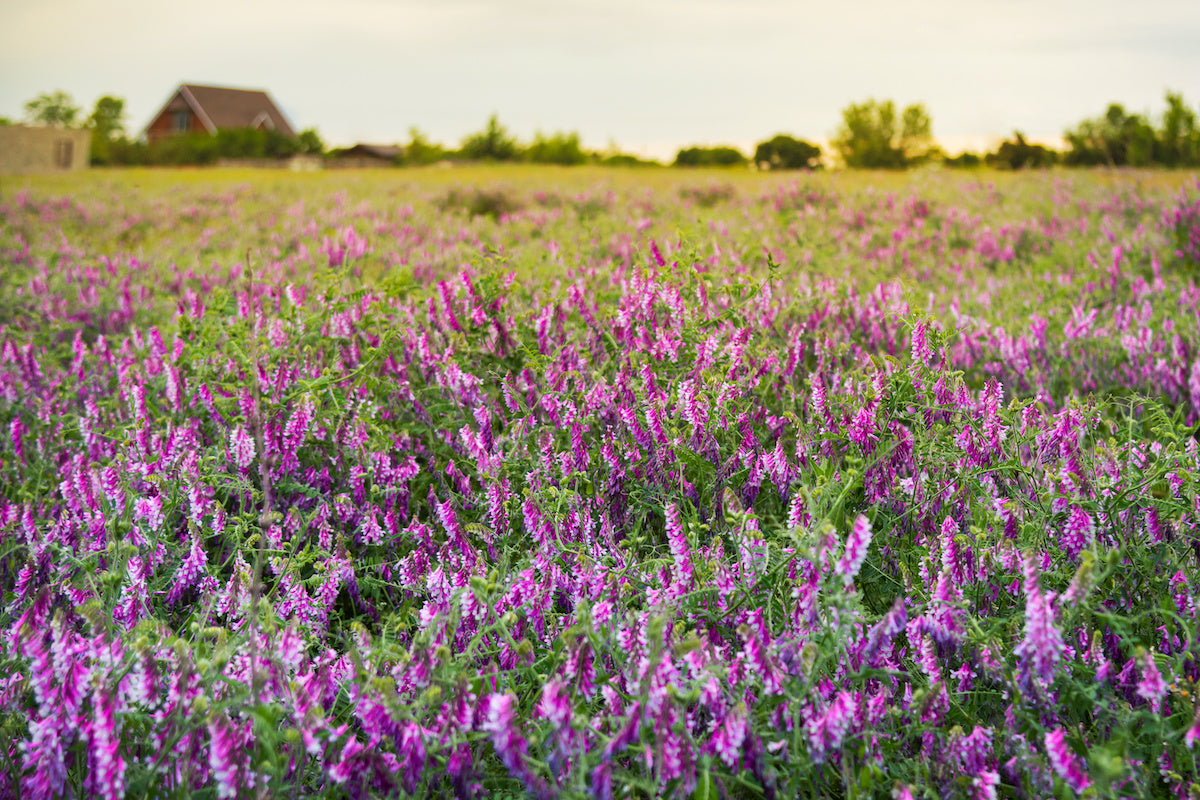This is a detailed daytime image of a vast, rural field dominated by tall, vibrant purple flowers that resemble sage or lavender, interspersed with green grass. The bright, varied shades of purple from light to dark create a dense, mesmerizing carpet. In the distant background, a red barn-like house with a gray roof stands out against a hazy, overcast sky, thick with white clouds. The scene is framed by lush green trees that line the area, creating a tranquil, picturesque landscape. The low-angle perspective of the photo accentuates the expansive field, entirely blanketed by these vertical blooms, evoking a sense of endless natural beauty.